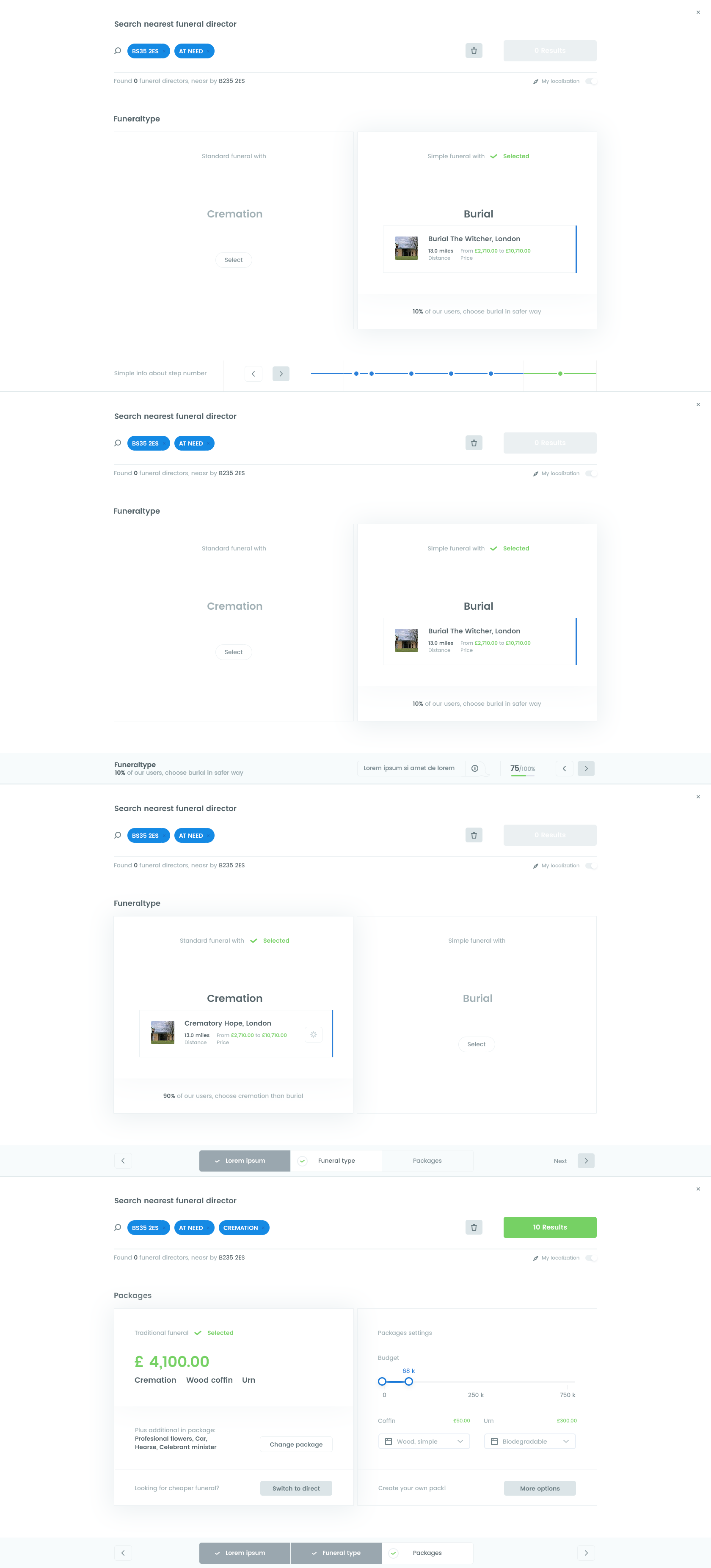Sure, here's a cleaned-up and detailed caption for the image described:

---

This digital interface showcases a search for the nearest funeral director, providing multiple options based on user preferences. On the left side, there are selection options for funeral types: a standard funeral, and a funeral with cremation. To the right, a menu highlights "Simple Funeral with Burial" as the selected option. "The Witcher London" is identified as a location 13 miles away, with an annotation stating that 10% of users choose burial as a safer way. Another location listed is "Crematory Hope London," also 13 miles distant, featuring a price of £4100 for cremation services. Additional details indicate options such as a wooden coffin and an urn for those opting for cremation. The interface provides a comprehensive overview of available funeral services and their associated options, aiding users in making informed decisions.

---

This caption aims to provide a clear and coherent description of all the key information presented in the image.